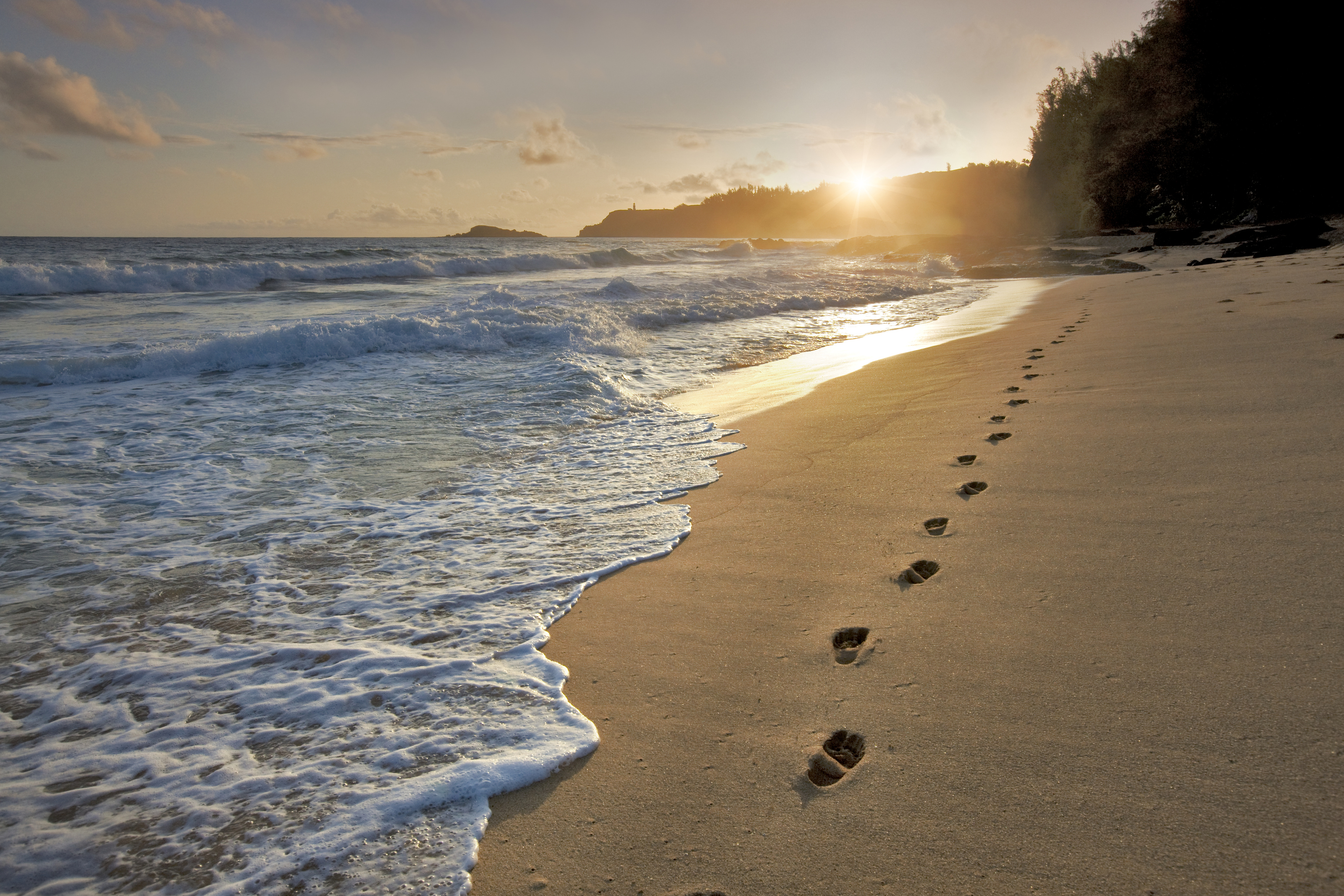The photograph captures a serene shoreline where foamy, white ocean waves crash gently onto the sandy beach. Imprinted in the sand, a trail of footprints follows the curve of the shoreline, running parallel to the water's edge. In the distance, a tree-lined elevation meets the ocean, adding a layer of natural beauty to the scene. Above the tree line, the sun is seen setting, casting a golden glow that permeates the image, enhancing the overall warm and inviting atmosphere. The sky is adorned with soft, white clouds, completing this picturesque coastal landscape.